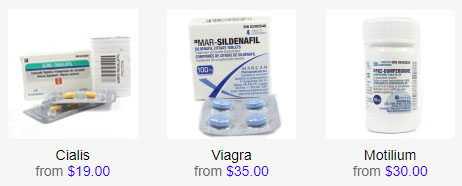This image depicts an online pharmacy specializing in medications for erectile dysfunction. Displayed are three different products: Cialis, Viagra, and a lesser-known drug called Motilium. 

Cialis is priced at $19 and comes in a small yellow pill packaged in a simplistic, tear-open packet. Viagra, known for its four distinctive blue pills, is available from $35. The image also provides its scientific name: Sildenafil. Motilium, which is less commonly recognized, is priced at $30 and is shown in a pill bottle, although the pill itself is not clearly visible.

This online store promotes easy access to these medications, reflecting the extensive advertising seen in various media.